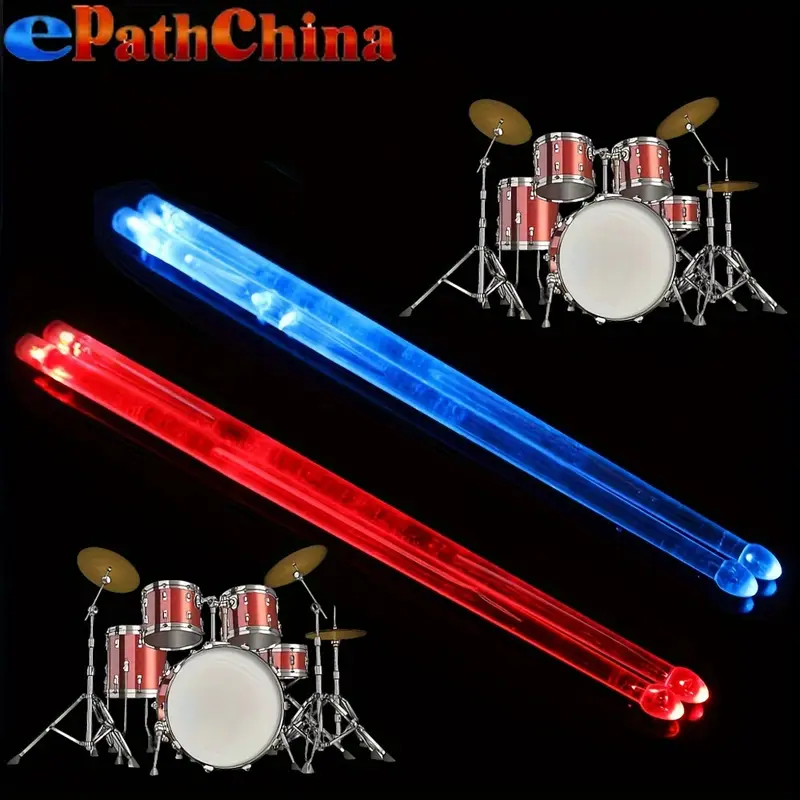This photograph showcases two red drum sets with shiny exteriors set against a black background. Prominently displayed in the top left corner is the ePathChina logo, with a lowercase 'e' in blue and 'PathChina' in red with a gradient pattern, styled in a serif font. Each drum set features a large white-topped bass drum and a set of three smaller drums along with golden-tinged metal cymbals tilted at an angle. In the center of the image, there are two pairs of glowing laser drumsticks placed below the drum sets. The blue glowing drumsticks are positioned in the upper portion, while the red glowing drumsticks are in the lower portion, adding a vibrant, illuminated effect to the overall composition.